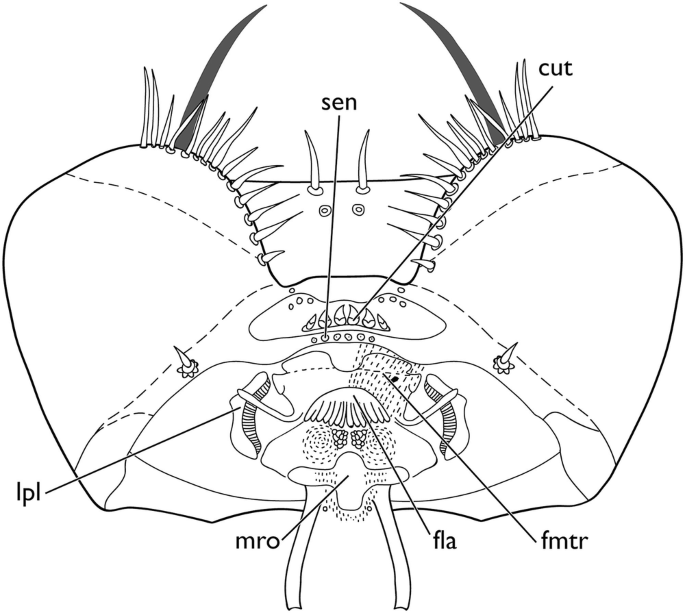The image depicts a detailed black and white line drawing, set against a white background, showcasing a close-up view of an object that appears to be an insect or perhaps an abstract organic form. The overall shape of the object is somewhat heart-like, with intricate details suggesting both texture and structure. At the top of the heart shape, there are fibers resembling feelers or antennae, indicative of some microscopic or minute creature, possibly a fly. Solid black lines emanate from various parts of the drawing, each labeled with acronyms: "SEN" at the top middle pointing to a small circle in the center, "CUT" on the right highlighting a sharp feature below, "LPL" on the bottom left indicating a curvy shape to its right, and other labels such as "MRO", "FLA", and "FMTR" pointing to further undefined parts. The image is clearly presented, with ample lighting that enhances its clarity, despite the complexity and the precise nature of its contents.